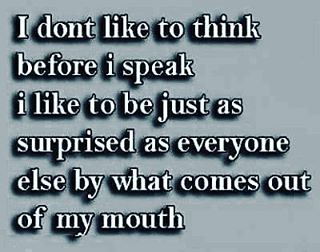The image features a solid gray background with a saying in white block letters, outlined in black and casting a shadow for added emphasis. The text reads: "I don't like to think before I speak. I like to be just as surprised as everyone else by what comes out of my mouth." The letters are predominantly lowercase, with the exception of the initial "I" which is capitalized.